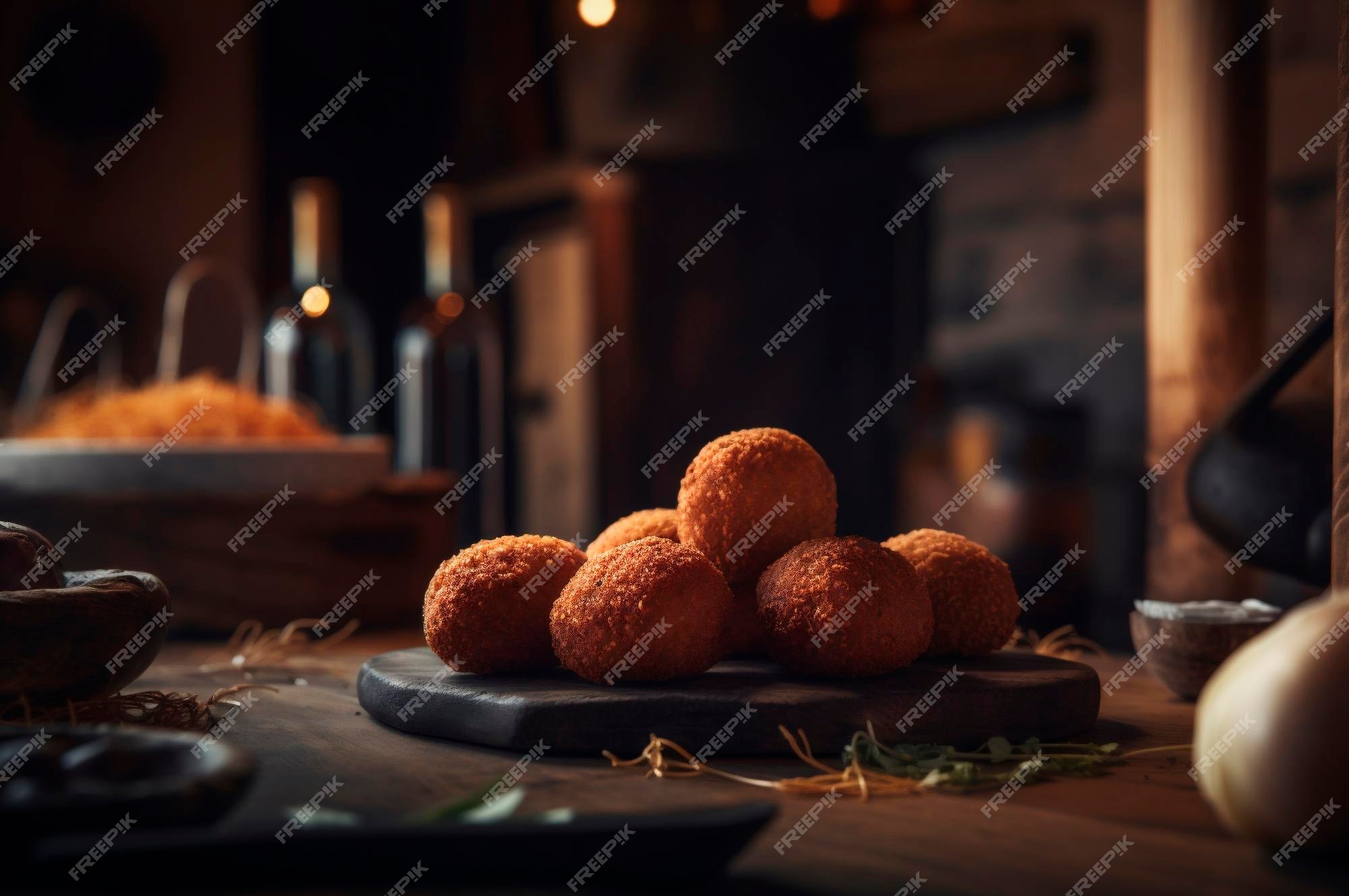This is a professionally styled photograph featuring a close-up of six round, golden-brown, breadcrumb-coated, fried food items, possibly resembling hush puppies or mozzarella balls. These items are meticulously arranged on a dark, black cutting board set atop a dark wooden table. The entire image is heavily watermarked with the text "Freepik," printed repeatedly in white letters diagonally from the bottom left to the top right, making detailed observation somewhat obscured.

The image background is blurred but suggests a dark kitchen or restaurant setting with dark wood accents. Notable elements in the blurred background include two bottles of wine and a silver plate with yellow rice to the left, as well as a possible coconut and a small wooden bowl or an avocado to the right. Additional decorations around the platter include some scattered greenery and an unidentified piece of fruit. Overall, the setting is warm and rustic, emphasizing dark brown tones and a cozy, inviting atmosphere.